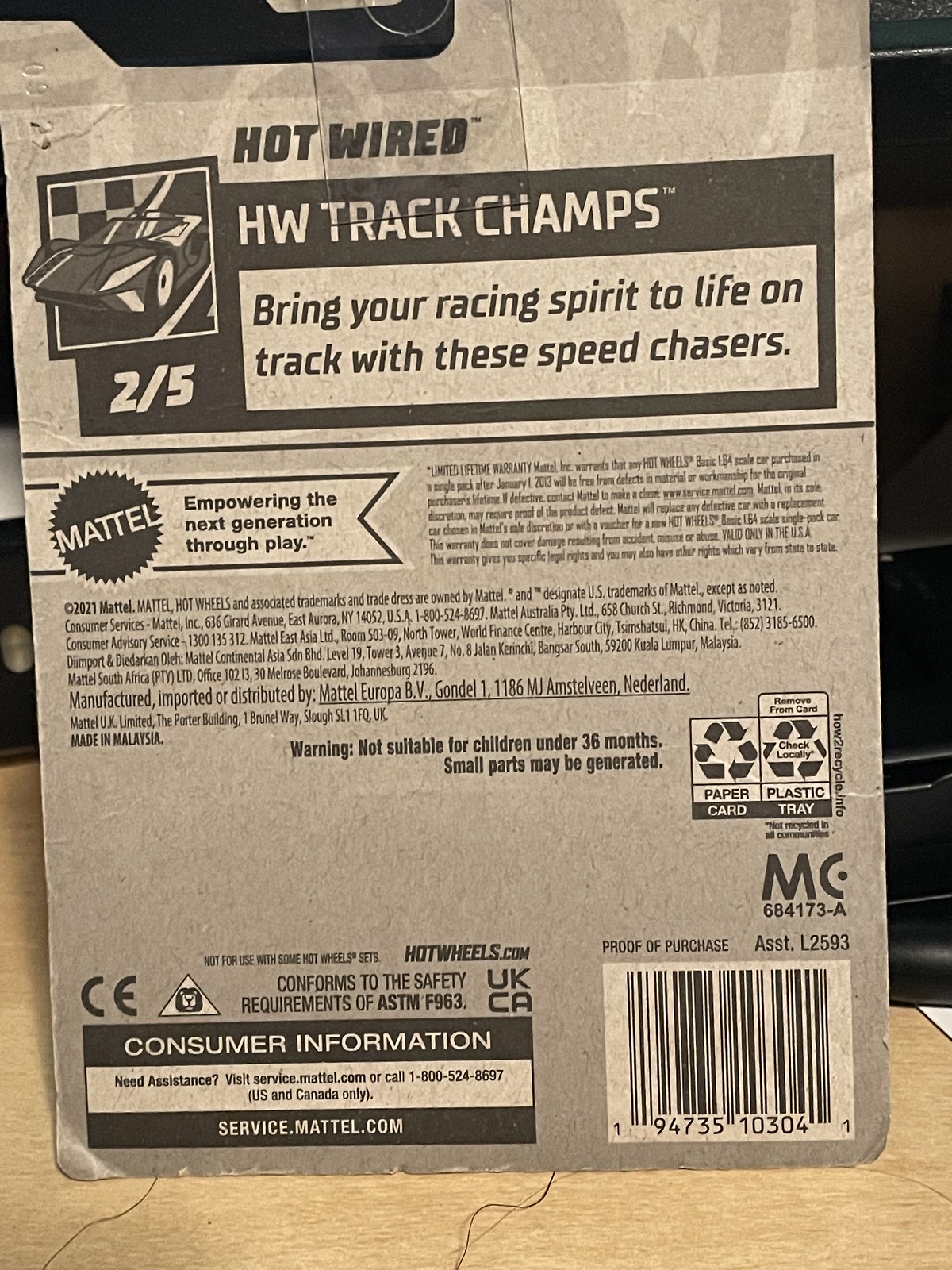The image depicts the cardboard backing of a Hot Wheels toy package. The cardboard has a pulpy, dingy gray texture. At the top left, there's a black and white illustration of a race car in a square tile with a checkered background. To the right of this illustration, the text "Hot Wired" appears in black, followed by "HW Track Champs" written in white. Below that, a promotional message in black reads, "Bring Your Racing Spirit to Life on track with these speed chasers." Toward the bottom middle in white text is the Mattel logo, accompanied by the slogan "Empowering the Next Generation Through Play" in black. Additional fine print provides company and consumer information, including a copyright notice “© 2021 Mattel” and warnings about small parts not being suitable for children under 36 months, as well as a barcode with the number "9473510304" below it. The display includes a cut-out at the top, typical for hanging on a rack in retail stores. The object is positioned on a brown desk with visible fibers that resemble black hair.